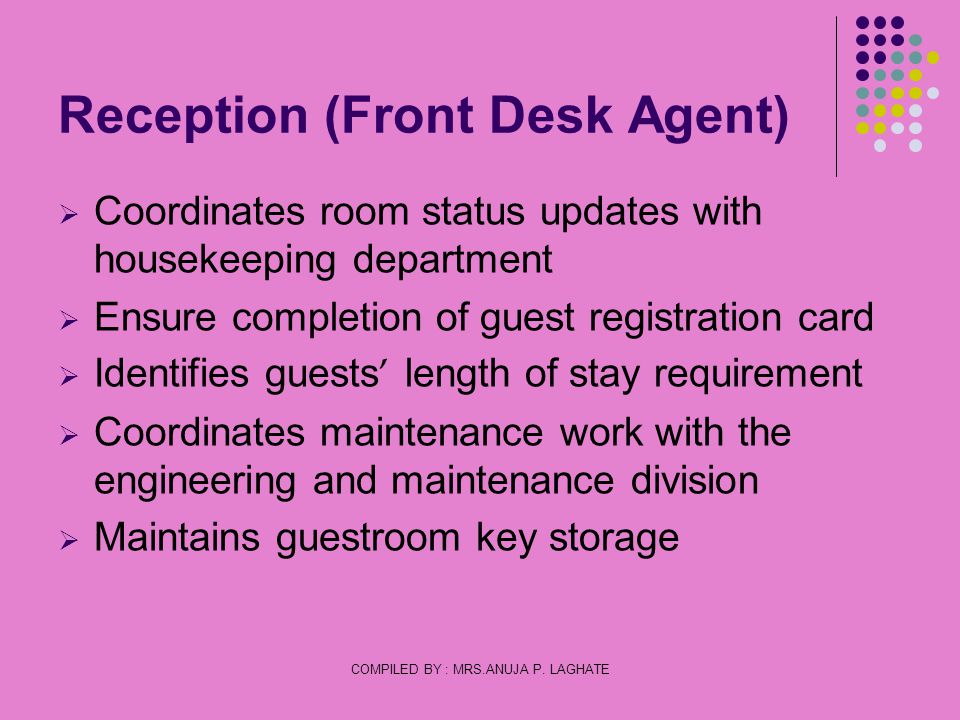The image features a text-centric presentation slide with a pink background. At the top, in dark purple text, it reads "Reception (Front Desk Agent)." The main content comprises five bullet points, each listed with a purple arrow. The bullet points in black text are: "Coordinates room status updates with the housekeeping department," "Ensure completion of guest registration card," "Identifies guests' length of stay requirement," "Coordinates maintenance work with the engineering and maintenance division," and "Maintains guest room key storage." In the bottom right corner, small black text states "Compiled by Mrs. Angela Pelagate.” A decorative vertical line adorned with a gradient of dots — transitioning from black to teal, greenish-yellow, and finally white — extends from the upper right corner, completing the design.